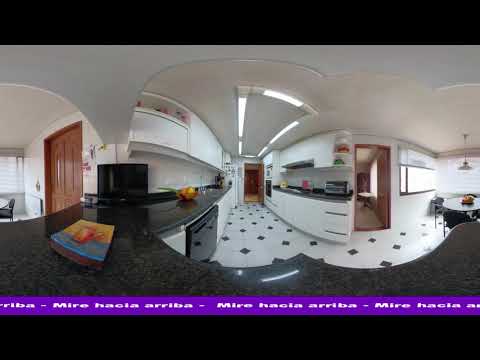The image presents an interior view of a house, primarily focusing on a kitchen setting captured with an extreme fisheye lens, giving it a panoramic, almost surreal look. The photo reveals a central hallway that leads through the kitchen, accentuated by a checkered tile floor with alternating large black and white squares. On the left side, there is a closed door, while an open door can be seen on the right and another one further in the background. The kitchen features countertops and a prep area, with a table and chair visible on the right side along with a hanging lamp above. Both the uppermost and bottom parts of the image are framed by black borders, just above which there is a blue stripe with text in Spanish reading "Miri Hacia Arriba" repeatedly, which translates to "Look Upwards". The overall color scheme of the image consists of black, purple, white, gray, blue, yellow, orange, tan, brown, and silver. Natural light enters the space through windows positioned on both the left and right sides, indicating it might be daytime. The combination of indoor lighting and outdoor natural light provides ample illumination for the scene.